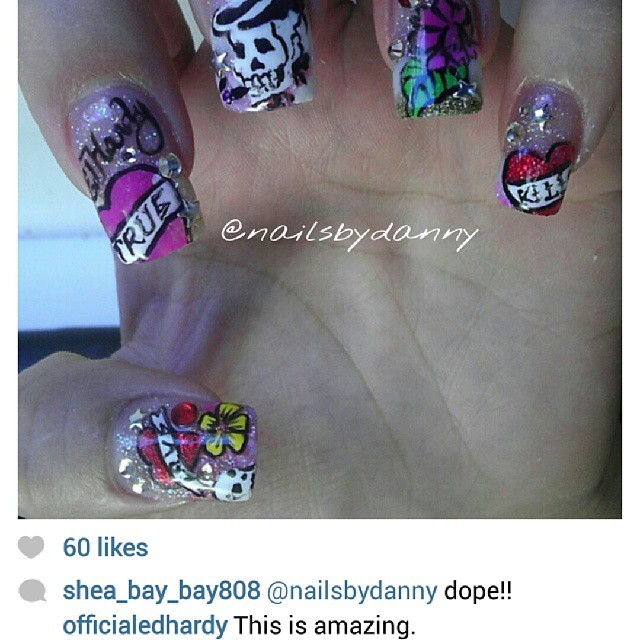A close-up image of a Caucasian person's left hand with their fingers folded inward to display intricately designed fingernails on each finger. The nails feature various Ed Hardy-themed designs on sparkly pink backgrounds. The thumb showcases a red heart with a white banner that reads "love," a small skull in the lower left corner, and a yellow flower in the right corner. The index finger has "Ed Hardy" written in black script with a pink heart and a "true" banner below it. The middle finger portrays a skull, appearing to smoke a cigar and has black and white hair. The ring finger is adorned with a large green leaf and a purple flower. The pinky features a red heart with a white "kills" banner. In the center of the palm, white text reads "@nailsbyDanny." Below the image, additional text includes a gray heart indicating "60 likes," a gray speech bubble with "Shea_bae_bae808 @nailsbyDanny," and the words "Dope!!" and "Official Ed Hardy wrote, 'This is amazing.'"